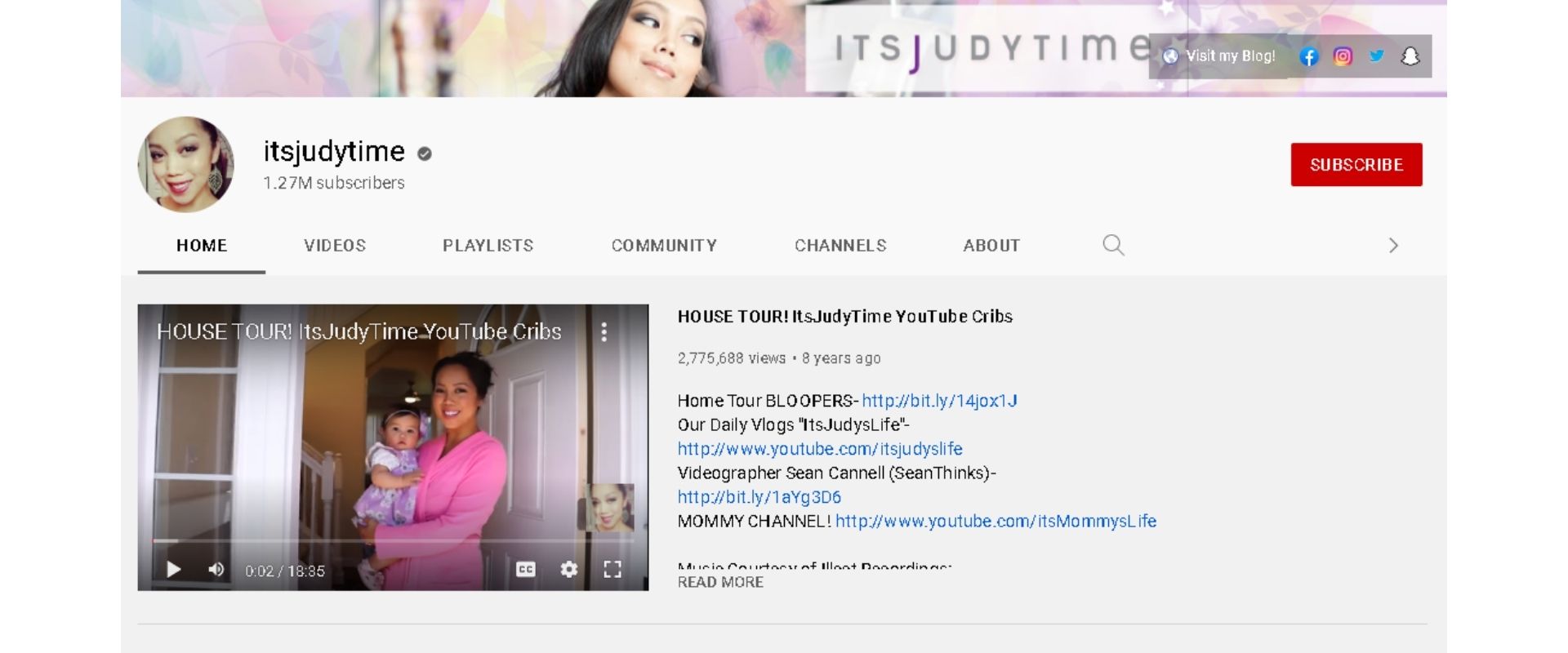This image is a detailed screenshot of a YouTube channel's homepage. At the top, there is a visually appealing header featuring a background adorned with pink and pale blue flowers. This also includes the face of a young female with dark hair and fair skin. To the right of her face, text reads, "It's Judy Time" with an invitation to visit her blog, alongside icons for Facebook, Instagram, Twitter, and what appears to be Reddit.

Beneath this header, there is a prominent red "Subscribe" button. On the left side of the screen, an image of the same young woman is shown within a round circle. Beside her image, the text "It's Judy Time" appears along with a verification checkmark and the subscriber count of 1.27 million.

At the bottom of the header, a horizontal menu extends from left to right with links labeled "Home," "Videos," "Playlists," "Community," "Channels," and "About."

To the left, a thumbnail image for a video titled "House Tour | It's Judy Time YouTube Cribs" is prominently displayed. The thumbnail features Judy herself, holding a small baby girl while standing in an open doorway.